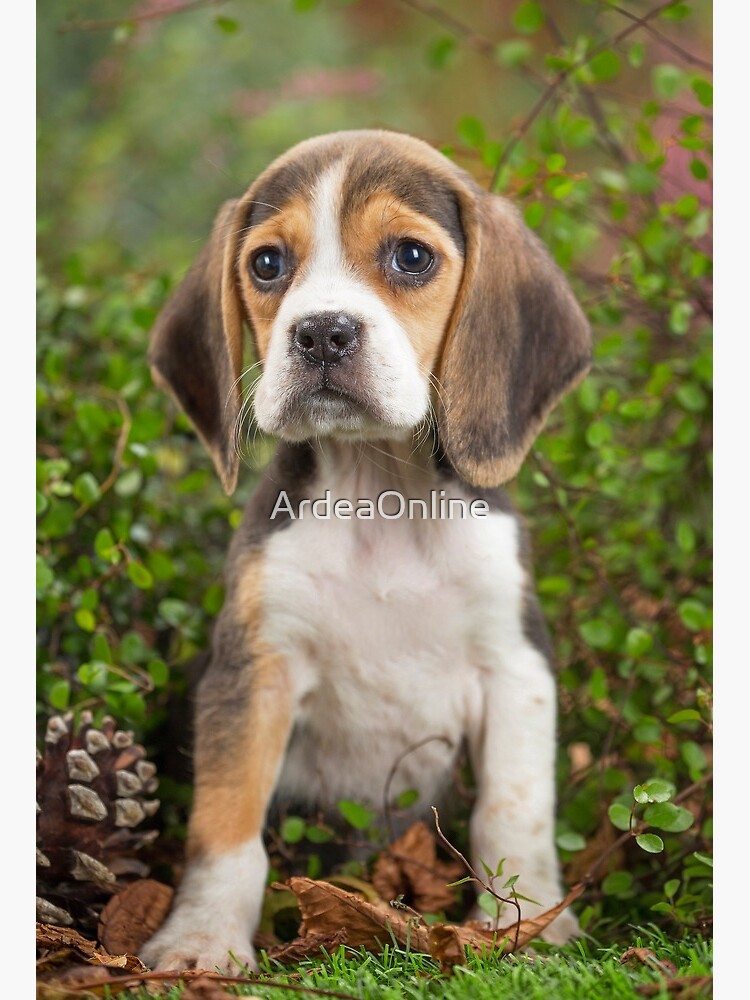In this beautiful and adorable photograph, there is a gorgeous beagle puppy sitting on a lawn in a garden. The puppy's coat is richly detailed: it has a white chest and paws, a white snout with a stripe running up its forehead, big brown eyes surrounded by light brown patches, and darker brown patches on its forehead, ears, and neck. The beagle's right front leg features a mix of white, reddish-brown, and dark brown coloring, typical of the breed. 

Behind the puppy, there's lush green foliage and brush, offering a vibrant natural backdrop, while the foreground includes some scattered brown leaves and a pine cone to the bottom left of the image. The focus of the image slightly blurs the background, emphasizing the beagle puppy's cute features. Prominently displayed in the middle of the picture is the text "ARDEA online," suggesting it might be from a stock photography website. This enchanting scene captures the essence of the beagle puppy's charm and the serene garden setting.